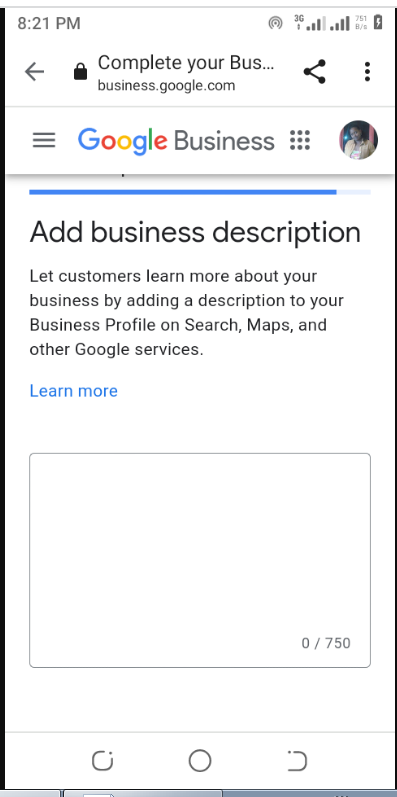The image appears to be a screenshot captured from a cell phone, displaying the Google Business website. In the top left corner, the time is shown as 8:21 p.m. On the top right, there are familiar status icons including a Wi-Fi symbol and a battery level indicator. Below the status icons, a partially visible message reads “Complete your biz...” next to a padlock symbol. This indicates the URL as business.google.com.

Directly beneath this header, the screen prominently displays the colorful Google logo followed by the label "Google Business." A bold blue horizontal bar spans across the width of the screen just below the label. The text below this bar prompts the user with "Add business description," encouraging them to enhance their business profile on Google Search, Maps, and other related services by adding a descriptive text. A clickable "Learn more" link in blue is situated underneath this instructional text.

The focal point of the screen is a large, empty rectangular text box intended for the business description, with a character count indicator at the bottom showing "0 / 750," highlighting the text input limit.

At the bottom of the screen, a navigation bar displays three icons: a rounded square on the left, a circle in the center, and a backward “C”-shaped symbol on the right, indicative of the typical Android navigation buttons for home, recent apps, and back functions.